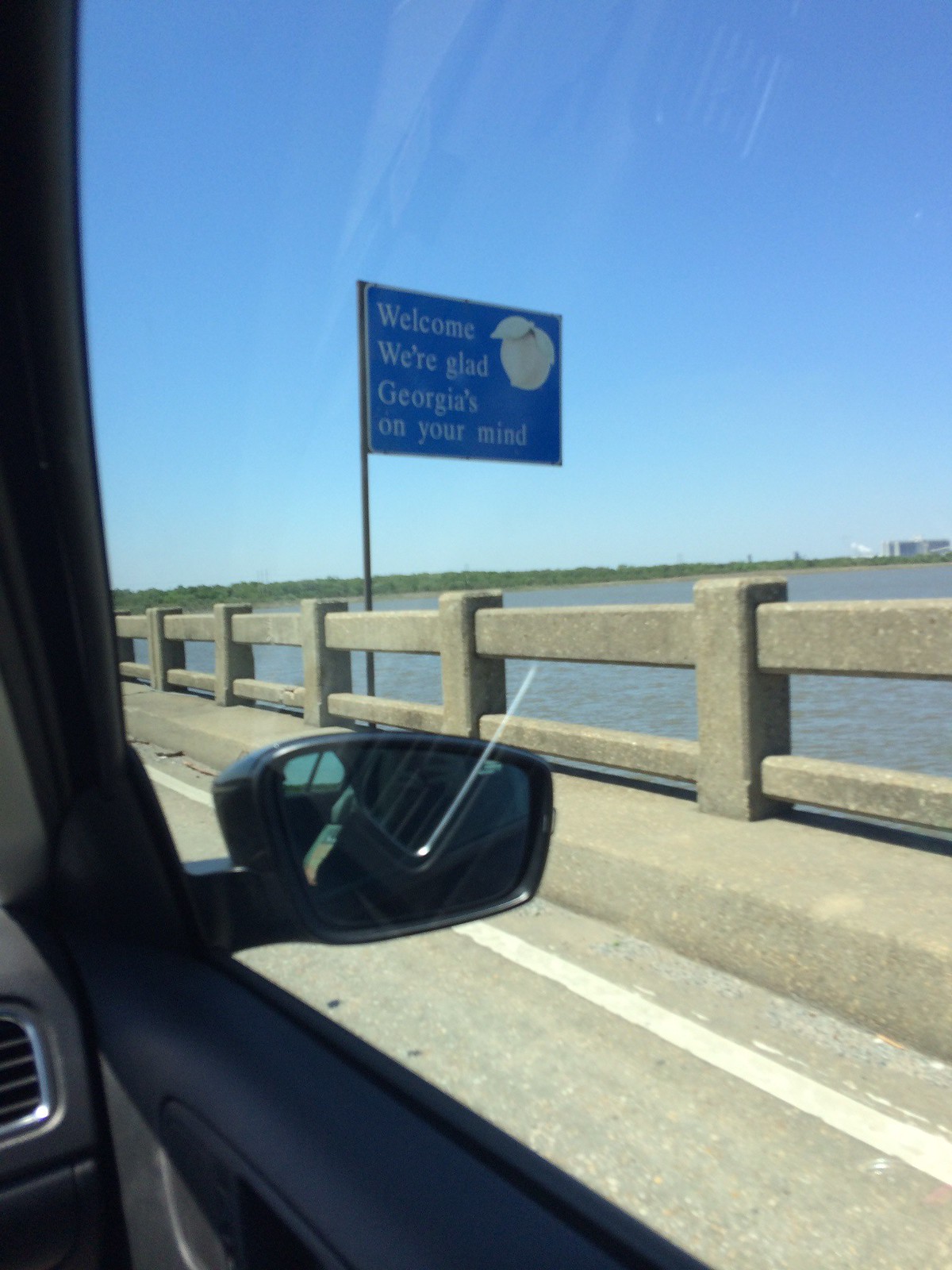A photograph taken from the passenger seat of a car captures a scenic view through the side window. The image showcases a concrete road lined with a white edge line, transitioning into a sidewalk with a thick stone railing consisting of rectangular shapes nested within each other. To the right of the stone barrier, expansive blue water stretches into the distance until it meets a green tree line, beneath a broad blue sky. Mounted on a pole beside the railing is a blue sign with white text that reads, "Welcome. We're glad Georgia's on your mind," accompanied by an image of a peach with two leaves in the upper right-hand corner. Inside the car, the gray interior is partially visible, including the side view mirror and the black-trimmed rearview mirror, with reflections on the window indicating that it is rolled up.